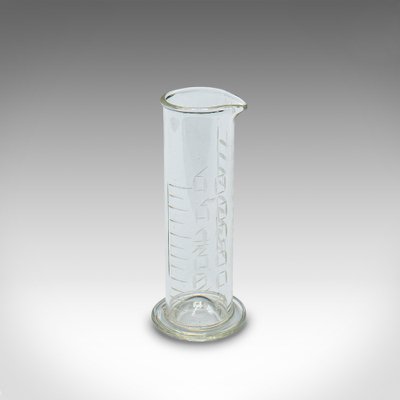The photograph is a black-and-white image featuring a cylindrical glass beaker prominently positioned at the center. The beaker, which appears to be of substantial and possibly older glass, stands upright on a clear, circular base. It has a small pouring spout oriented towards the right. Along the left side of the beaker are horizontal measurement lines, resembling those on a ruler, with numbers inscribed from 0 to 6, although other etchings or text are present but not clearly legible. The background of the photograph transitions from a darker gray at the top to white at the bottom, with the bottom corners showing a subtle gradient back to gray.